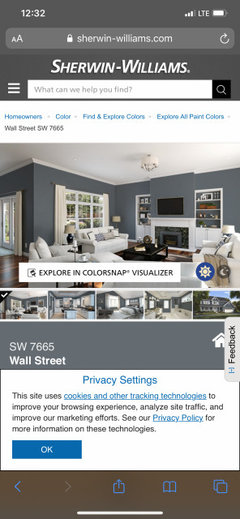A screenshot taken on a smartphone displays the Sherwin-Williams website. At the top of the screen, the time reads 12:32, accompanied by network coverage bars, LTE signal indicator, and a battery icon. The browser’s address bar shows the URL "SherwinWilliams.com."

Below this, "Sherwin-Williams" appears in bold, white, capitalized letters. A search bar prompts, "What can we help you find?" followed by navigation options labeled "Homeowners," "Color," "Find and Explore Colors," and "Explore All Paint Colors." The wall color "Wall Street SW 7665" is noted.

The main section of the screenshot features a photo of a stylish living room. The walls are painted in a dark gray color. The furnishings include white couches and chairs. A fireplace with a white mantle holds a flat-screen TV mounted above it. Flanking the fireplace are white bookcases. A white banner across the photograph reads, "Explore in Color Snap Visualizer." 

Icons of a blue circle with a yellow sun and a black circle featuring a white crescent moon are visible. Below, a dark gray banner, matching the room's wall color, displays the text "SW 7665 Wall Street."

At the bottom, privacy information is provided, explaining the use of cookies and other tracking technologies to enhance browsing experience and improve marketing efforts. It advises readers to consult the privacy policy for more details. A blue rectangle with the word "OK" in white lettering offers users the option to consent.